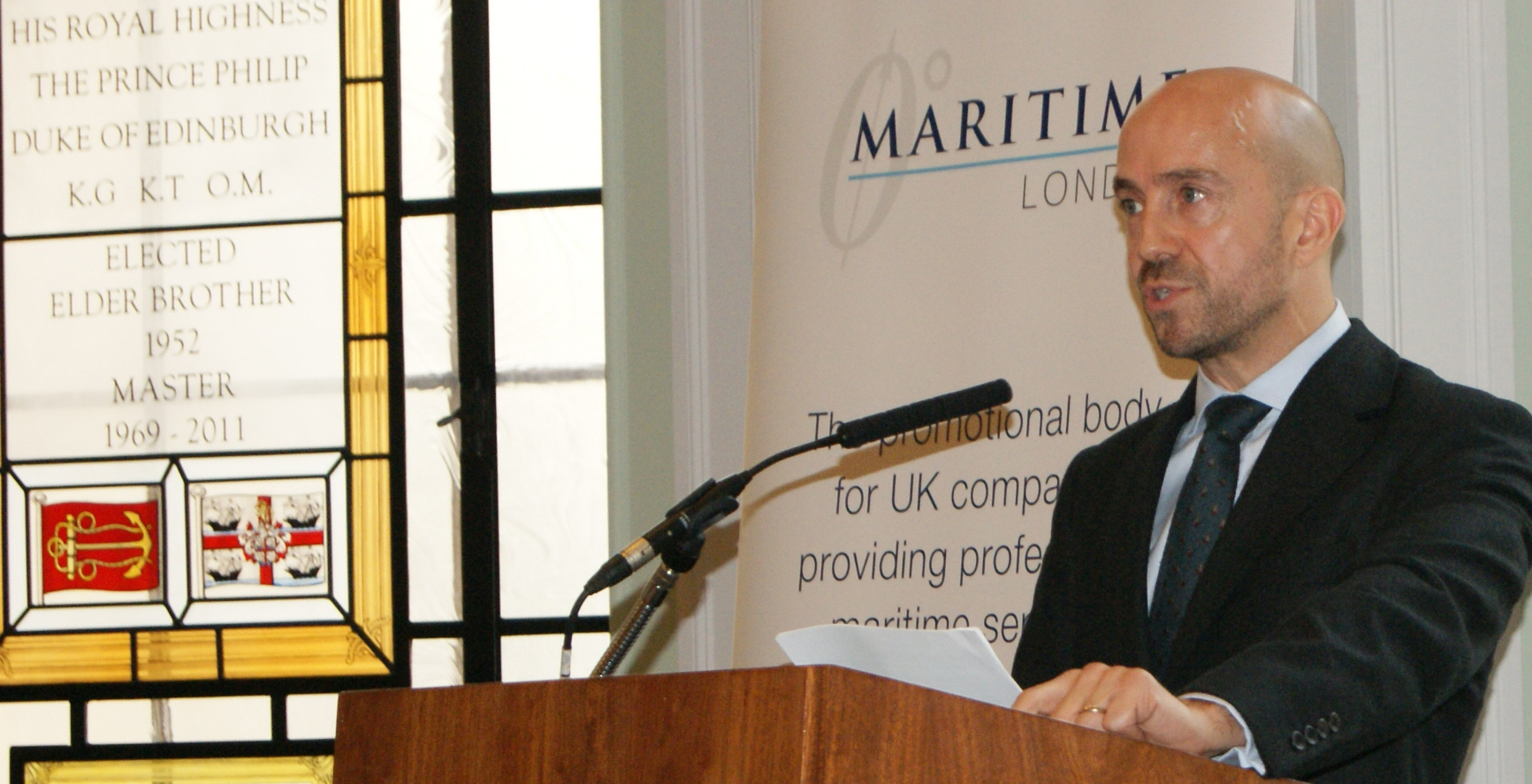In a detailed image of a man delivering a presentation at a conference, he stands behind a wooden podium equipped with a long, skinny microphone directed toward him. The gentleman, who sports a shaved head and a 5 o'clock shadow stubble, is dressed impeccably in a white collared shirt paired with a dark blue tie and blazer. Holding a piece of paper in his left hand, he addresses the audience with a backdrop featuring the words "Maritime London." The backdrop text, partially obscured by his figure and the microphone, mentions "the promotional body for UK companies" before trailing off. Flanking him on the left is a stained glass window with a gold border, inscribed with "His Royal Highness the Prince Philip, Duke of Edinburgh, KGKTOM, elected elder brother 1952, master 1969-2011." Below this inscription are two artistic panes: one showcasing a red flag with a yellow symbol and the other a white flag adorned with a red cross and additional blue and red elements.